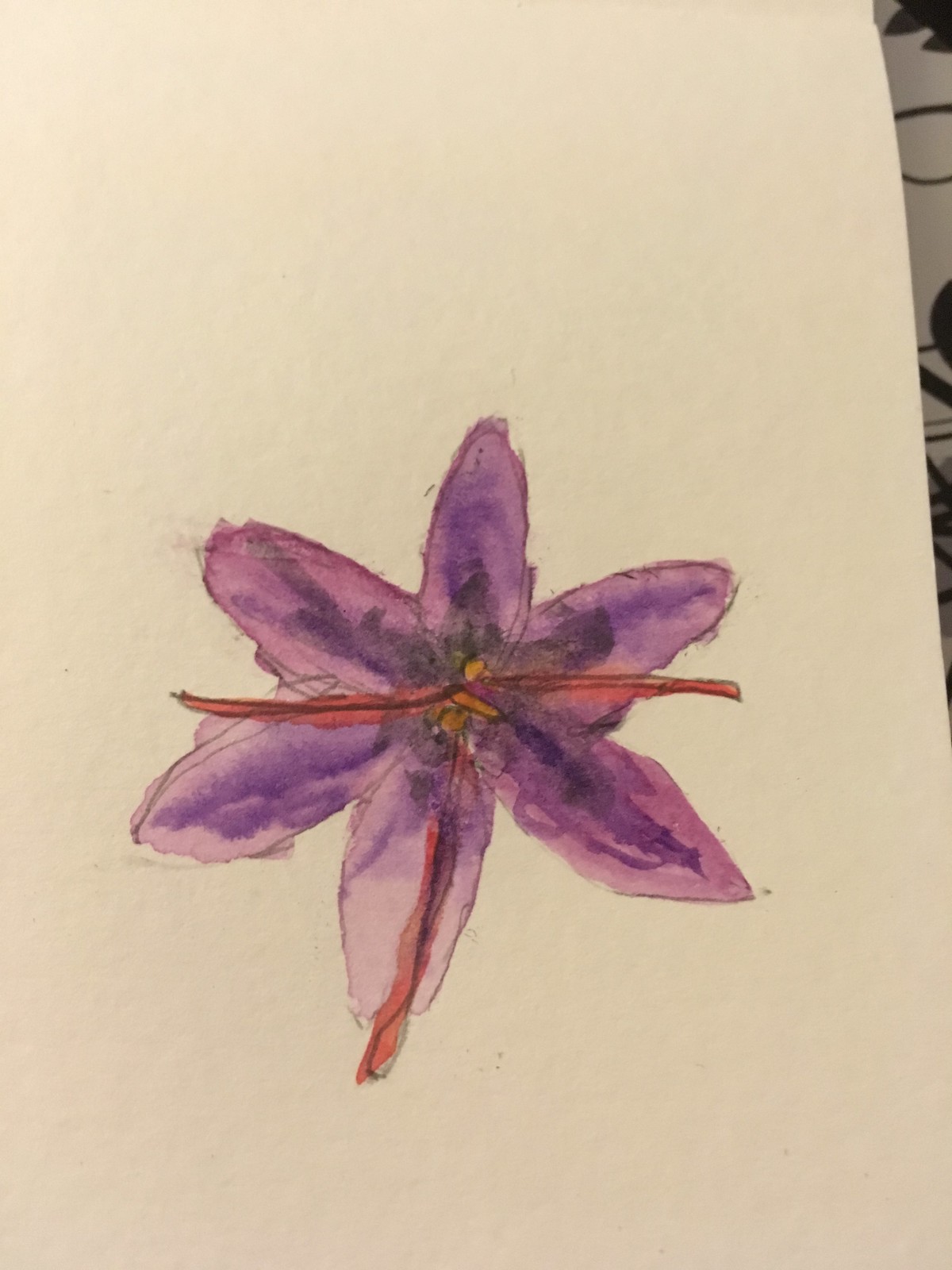This vertical rectangular watercolor painting features a six-petal purple flower prominently centered on an off-white or cream-colored paper, possibly from a pad. The flower's petals are delicately shaded, with a gradient transitioning from a lighter pinkish-purple at the edges to a darker purple toward the center. The central part of the flower is accentuated with darker purple and a touch of yellow. The flower is further detailed with pencil marks still visible beneath the watercolor, hinting at an initial sketch. Three thin, red lines, outlined in black, intersect the flower—two horizontally and one vertically down a petal—adding a distinctive and contrasting element. The background shows hints of a brown design in the top right corner, partially bordering the predominantly off-white canvas. The overall impression is of a piece created by someone exploring watercolor techniques, capturing the flower's natural beauty with a learning hand.